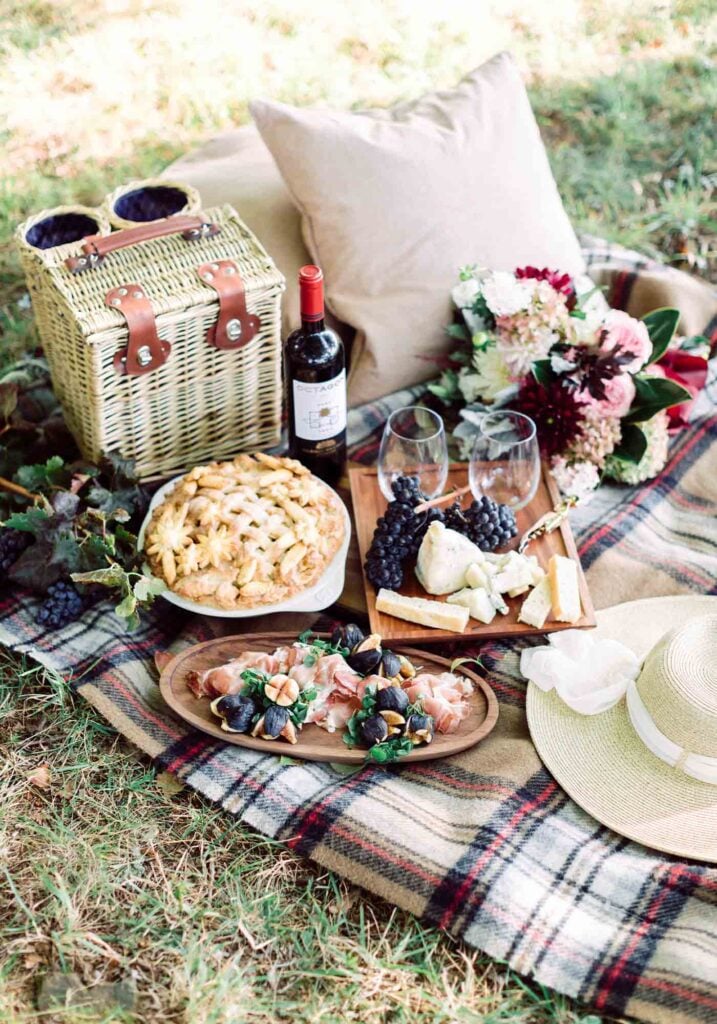The vibrant and inviting photograph captures a picturesque outdoor picnic setup on a field of mixed green and brown grass, bathed in sunlight. A plaid blanket with tan, red, and black stripes is elegantly spread out, adorned with carefully arranged picnic essentials. At the bottom right, a stylish off-white lady's hat with a ribbon adds a touch of charm. Two soft, beige pillows enhance the cozy atmosphere. 

The picnic spread features an array of delectable treats: a wooden platter with fresh figs and slices of prosciutto, another wooden tray holding juicy grapes, assorted cheeses, two empty wine glasses, and a bottle of wine, ready to be served. An apple pie with a lattice crust, set in a white dish, tempts from the side. Nearby, an oval wooden platter presents more culinary delights, possibly including shrimp or vegetables. In the background sits a wicker basket containing two additional bottles of wine. 

Adding to the picturesque scene, a bouquet of flowers and vines laden with grapes embellish the left side of the blanket. The entire setup exudes a sense of tranquility and warmth, inviting viewers to imagine themselves enjoying this idyllic picnic.